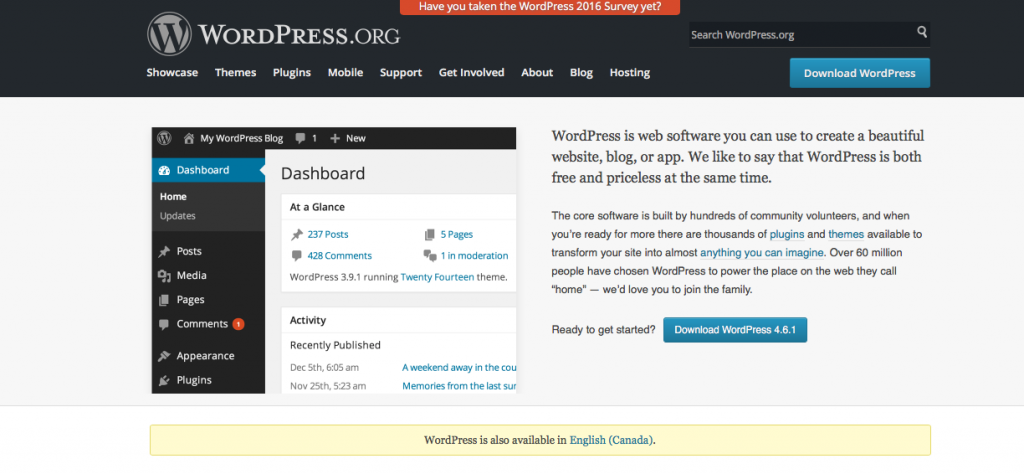A detailed screenshot of a user navigating the WordPress.org admin panel. The user is currently on the WordPress.org homepage, which features a dark gray header displaying various menu options including Showcase, Themes, Plugins, Mobile Support, Get Involved, About, Blog, and Hosting. Prominently at the top center, an orange drop-down banner inquires, "Have you taken the WordPress 2016 survey yet?" 

On the right side of the header, there's a search field labeled "Search WordPress.org," next to a light blue button. In the lower right corner, a similar button stands out with the text "Download WordPress" in white font against a light blue background.

Below the header, the main content area transitions to a clean, white dashboard centered within the page. The dashboard isn’t as wide as the dark gray header. The header of the dashboard reads "My WordPress Blog" with a notification icon indicating a new message. The main navigation menu running down the left sidebar is highlighted, with "Dashboard" selected in blue. Other visible options include Home, Updates, Posts, Media, Pages, Comments (indicating one unread comment), Appearance, and Plugins.

Within the "Dashboard at a Glance" section, the user can see a summary displaying 237 posts, 428 comments, five pages, one comment in moderation, and the active 2014 theme. Recent activity is noted under the "Activity" section, showing recent posts: "A Weekend Away in the Country" published on December 5th at 6 a.m. and "Memories from the Last Summer" published on November 25th at 5:23 a.m.

To the right of this content, an informative section explains WordPress, describing it as web software for creating beautiful websites, blogs, or apps, and emphasizing its dual nature of being both free and priceless. At the bottom of this section, a blue button states "Ready to get started? Download WordPress 4.6.1" inviting users to take the next step.